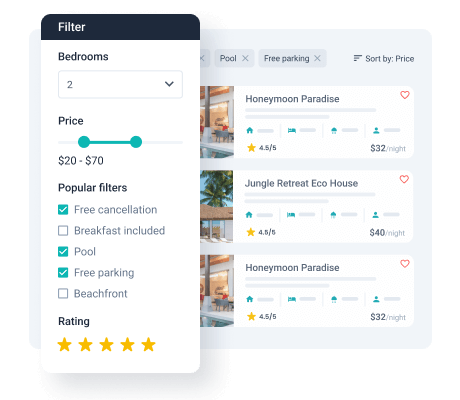The image features a detailed view of a travel application's filtering interface used for searching accommodations. On the far left, there is a single column displayed, featuring a pop-up screen with a black title bar that reads "Filters." Below the title bar, there is a section for bedroom preferences, allowing users to select the number of bedrooms via a box currently displaying the number two.

Further down is a green-colored price slider bar with two adjustable dots on either end, enabling users to set a price range from $20 to $70. Below the price slider, there are various popular filter options, each represented by a square box that can be tapped to activate. When selected, these boxes turn green with check marks inside. In this instance, the filters for "Free Cancellation," "Pool," and "Free Parking" have been chosen.

Continuing down, the rating section allows users to select the desired star rating for accommodations, with the current selection being five yellow stars. This column partially obscures approximately half of the actual search results behind it.

Beneath the filter column, the search results begin with accommodations that match the selected criteria. The results include "Honeymoon Paradise," "Jungle Retreat Eco House," and once again, "Honeymoon Paradise." Each listing displays its star rating and price, highlighting amenities such as a pool and free parking. The interface also offers a "Sort by Price" feature, allowing users to organize the results based on their budget preferences.